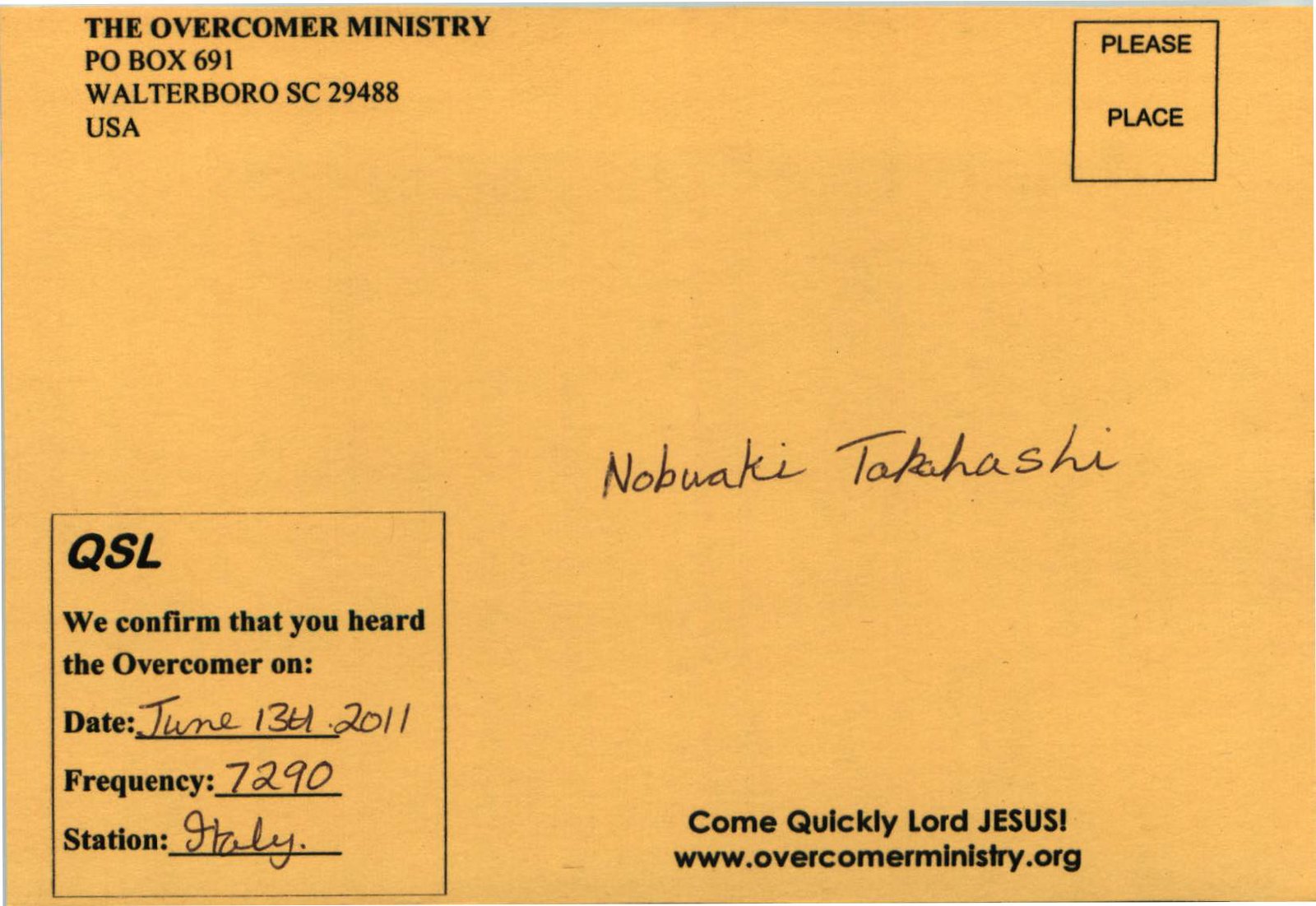This image shows the back of an orange-colored postcard associated with the Overcomer Ministry. In the upper left corner, printed in black, is the address: "Overcomer Ministry, P.O. Box 691, Waterboro, SC 29488 USA." In the upper right corner, there's a square outline with the instruction "Please Place" indicating where to put the stamp. In the middle of the postcard, there's a handwritten signature that reads "Nabuki Takahashi." The bottom of the card features the phrase "Come quickly, Lord Jesus" followed by the website "www.overcomerministry.org" printed in black. On the lower left side, a boxed label with "QSL" confirms receipt of transmission from the Overcomer Ministry, detailing the reception date as January 13, 2011, on frequency 7290 from a station located in Italy.